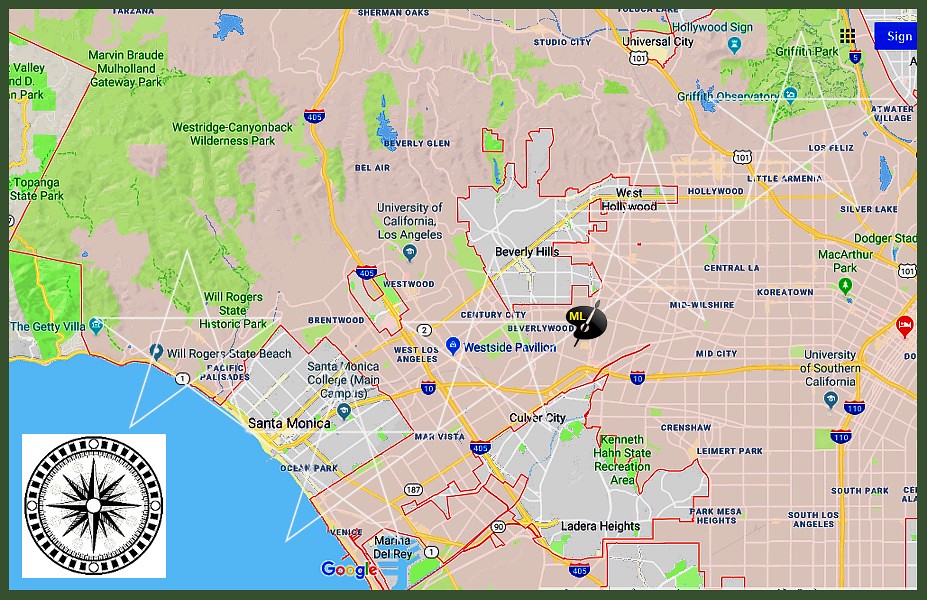A detailed photograph of a map depicts the intricate layout of the West Coast region of California, highlighting the Los Angeles area. The blue expanse of the Pacific Ocean frames the left side of the map, clearly illustrating the coastline. Key interstates, such as the 405, 10, and 110, are prominently marked in yellow, weaving through the various urban zones.

Numerous cities are denoted in gray, including West Hollywood, Beverly Hills, Santa Monica, Culver City, Ladera Heights, and Marina Del Rey, with the latter uniquely highlighted in blue. Green areas, representing parks or significant recreational spaces, are interspersed throughout the urban landscape. Notable parks such as Griffith Park, MacArthur Park, Marvin Braude Mulholland Gateway Park, and Westridge Canyonback Wilderness Park are clearly labeled, along with landmark sites like the Getty Villa.

Additional neighborhoods are indicated with their respective names, though individual road names are not shown. These areas encompass Brentwood, Westwood, West Los Angeles, Mar Vista, Beverlywood, Century City, Mid-Wilshire, Koreatown, Crenshaw, Leimert Park, Park Mesa Heights, South Los Angeles, and South Park. The overall map offers a comprehensive and detailed view of this iconic region, blending natural landscapes with the dense urban sprawl.